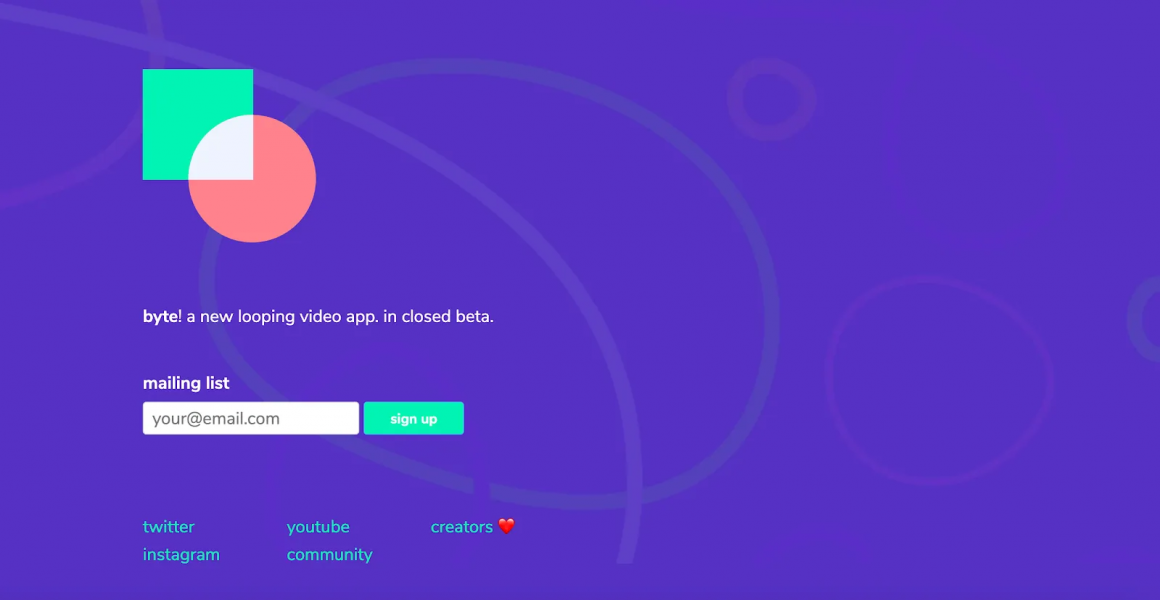This is a detailed screenshot from a website or app named Byte, a new looping video platform currently in closed beta. The page prominently features a call-to-action encouraging visitors to join a mailing list by inputting their email addresses, presumably to receive updates or be notified when the app officially launches. The design includes links to Byte's social media accounts, including Twitter, YouTube, and Instagram, as well as additional links labeled "Community" and "Creators," the latter adorned with a heart emoji. The logo, a minimalist design, consists of a green square and a red circle that overlap at the bottom right and top left corners, respectively. The entire layout is set against a subtle purple background, faintly decorated with abstract circles and ovals, giving the page a modern and visually appealing aesthetic.